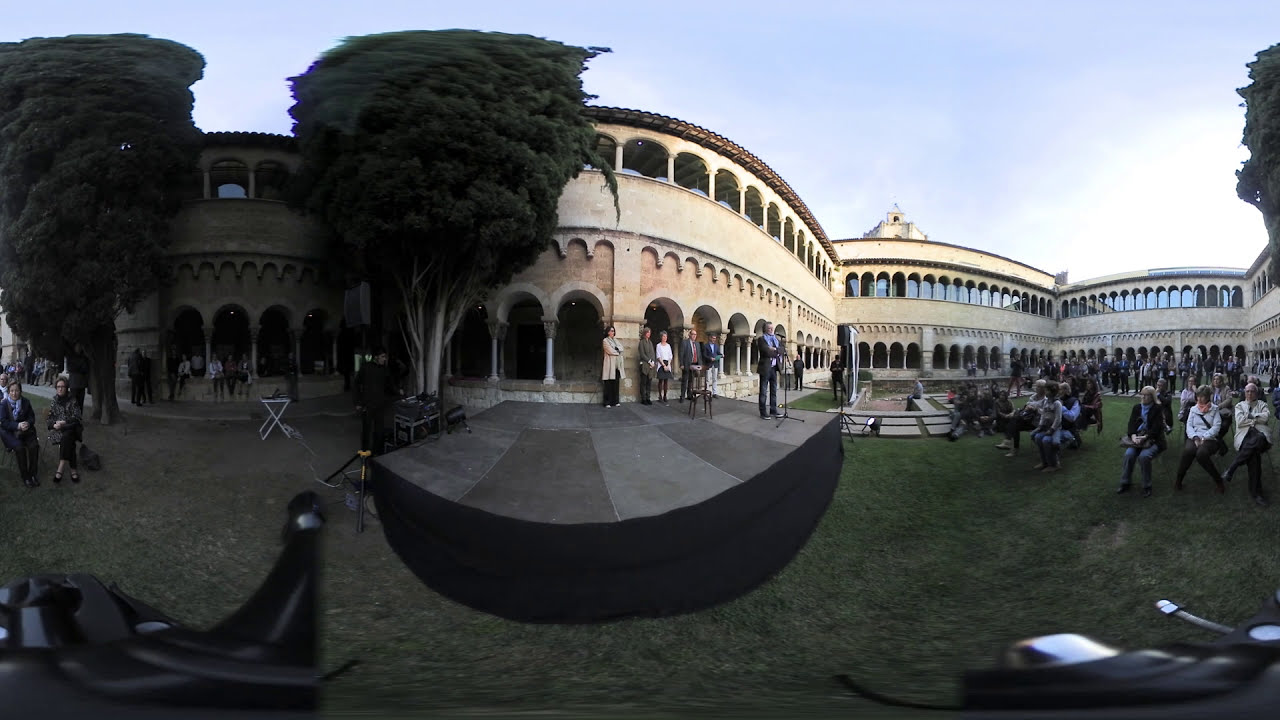This image captures a bustling outdoor gathering taking place in a spacious courtyard on a university or college campus. The scene is dominated by a massive, two-story building with light brown brick or stone walls, featuring numerous arches on both floors. The first-floor arches are open, while the second-floor arches serve as windows with glass. This extensive, horizontally stretched-out structure is adorned with ornate decorations and showcases an open balcony with windows at the top. 

In the courtyard, a significant crowd is gathered on the well-maintained green grass, with many attendees seated on chairs, listening to a speaker who is positioned on a raised stage. This stage has a gray floor and a black front and is equipped with microphones. The speaker, dressed formally, stands at the edge of the stage, while other individuals, also in smart dress, stand at the back corner of the platform. There are tables on the stage, indicating a formal event. 

On the left side of the image, two large trees provide a natural frame next to the expansive building. The sky above is a clear blue, adding to the vibrant atmosphere of the event. The entire setting is abuzz with activity, capturing the essence of a lively, outdoor event on a picturesque day.